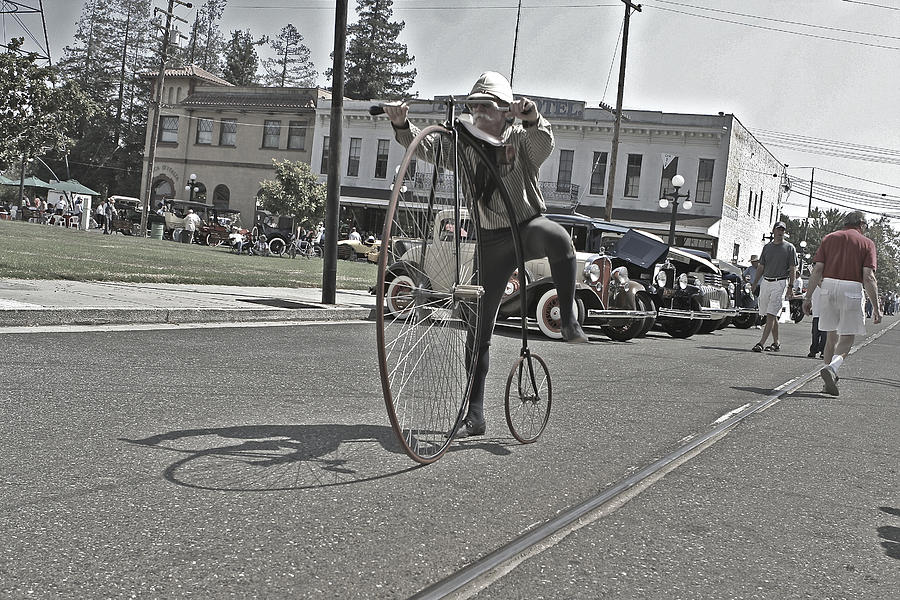A vivid outdoor daytime photograph captures a lively vintage car exhibition set on a gray paved road featuring a prominent centerline. The foreground spotlights an elderly man with a distinguished white mustache, dressed in a gray cap, a blousey gray-and-white shirt, and gray pants. With his right leg grounded and his left leg raised in mid-motion, he is preparing to mount an old-style bicycle, characterized by an enormous front wheel, approximately five to six feet tall, and a much smaller back wheel, just knee-high. His hands grip the handlebars, which stretch above shoulder level.

Surrounding this focal scene, a group of people mingles on the right side of the road, dressed casually in shorts and t-shirts, further adding to the nostalgic charm. Throughout the scene spans a row of vintage cars, reminiscent of the early 19th century, lined along the street and curving left around the corner. The background showcases a blend of historic stone buildings, lush green fields, and scattered trees under a slightly cloudy sky, with overhead electrical poles and wires providing a touch of quaint authenticity to the setting.